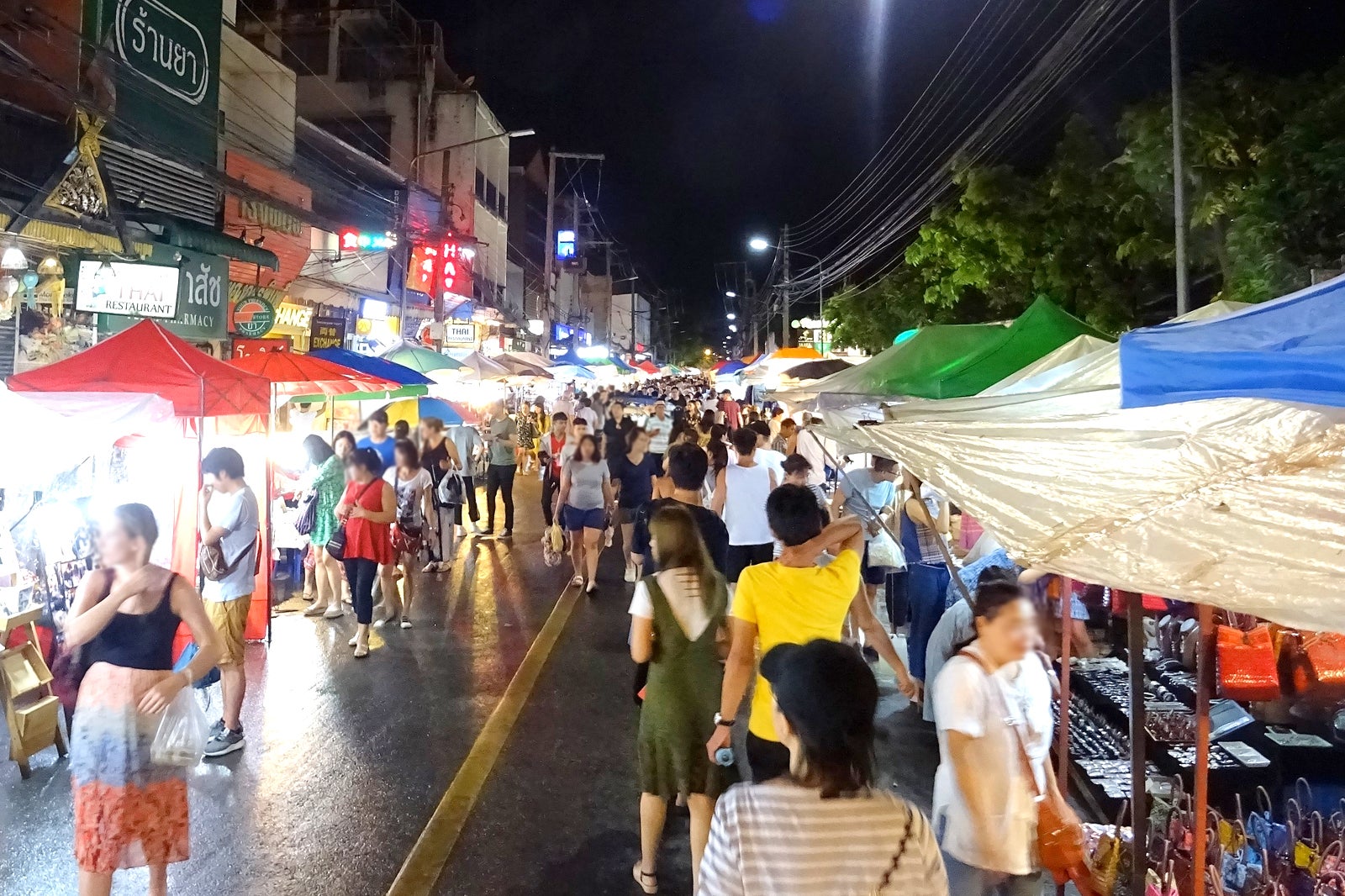In this nighttime urban scene, a bustling street market is filled with activity. The crowded market features numerous vendors' booths, each adorned with colorful canopies in shades of blue, green, beige, red, white, and orange. This varied array of umbrellas stretches into the distance on both sides of the street, creating a vibrant atmosphere. On the right, vendors are selling jewelry and bags of different colors, with many people perusing their wares. The left side reveals more stores connected to white buildings, also under multicolored canopies. Electrical wires crisscross overhead, illuminated by white street lamps. The market stalls are set up along a street marked by a yellow line in the middle, where the lively crowd navigates between shopping and exploring. The scene suggests a fair or farmer's market, capturing a snapshot of urban life against the dark night sky.